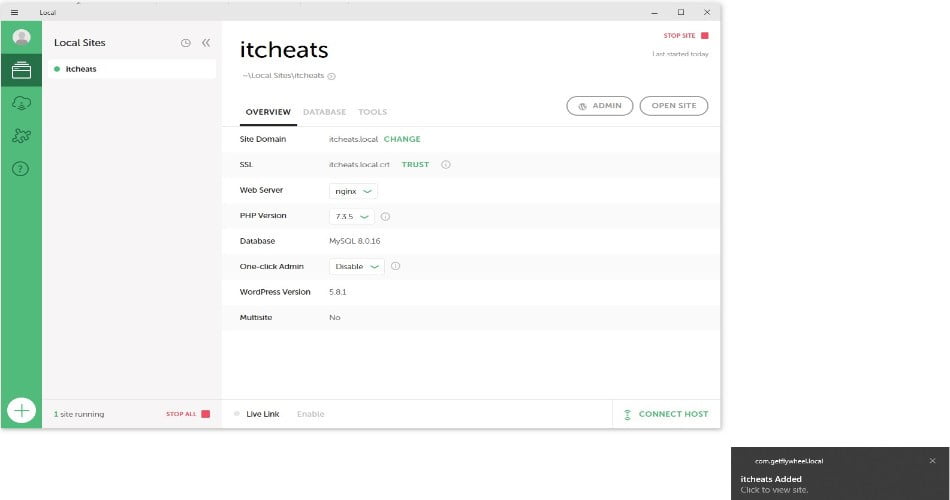The image is a screenshot of a "Local" window on a Windows OS. The window does not appear to be from a website but rather a local application. The title of the window is "Local" and it features a standard Windows interface. On the left-hand side, there is a vertical green bar with several icons, each representing different functionalities. The icons include a person inside a circle, a box, a cloud, a jigsaw puzzle, and a question mark. At the bottom of this bar, there is a plus icon, likely for adding additional items.

Adjacent to the green bar is a gray column labeled "Local Sites." Below this label, a green dot is shown beside the text "IT Cheats," indicating an active status. The main area of the window provides an overview of "IT Cheats" under the "Local Sites" section. This area displays various technical details such as site domain, SSL, web server, PHP version, database, one-click admin, WordPress version, and another unclear item.

In the upper right corner, there are two buttons labeled "Admin" and "Open Site." Above these buttons, a red box with red text saying "Stop Site" is visible, indicating that the site is currently running and can be stopped.

Overall, the screenshot appears to be a management interface for local websites, providing tools and information for site administration.